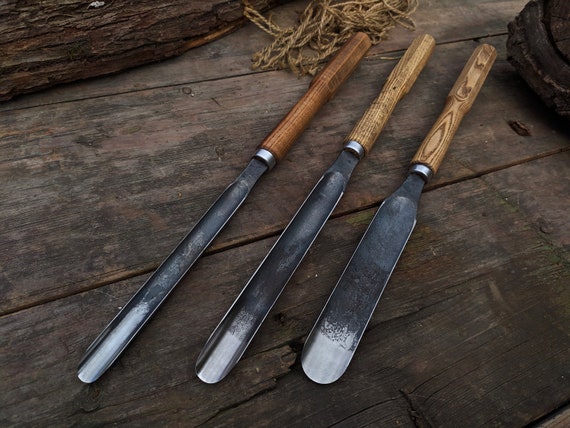The image displays three garden or chisel-like tools laid side by side on a dark wooden surface. Each tool features a shiny black metal blade that progressively increases in width from left to right. The tool on the left has the thinnest blade, resembling a long slender butter knife with turned-up sides forming a small trough. Its handle is dark brown. The middle tool has a slightly wider blade and a light brown wooden handle. The third and final tool has the widest blade, more rounded, with a handle that includes dark brown rings, giving it a distinct appearance compared to the other two. All three tools feature wooden handles, though the shades of brown vary. In the top left corner of the image, part of a tree trunk rests horizontally at a diagonal, adding a rustic element to the scene.